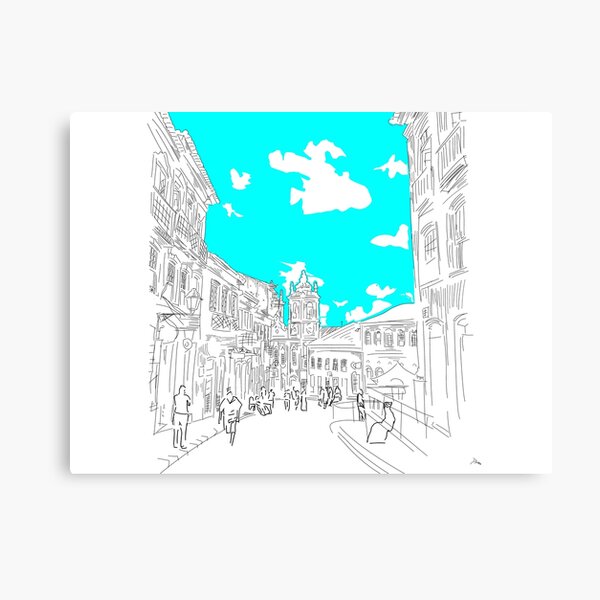The artwork is a black and white sketch of a bustling city street, set against a solid white background. This dynamic scene features buildings on both sides of a winding street, intricately outlined with an eye for perspective. The buildings, while merely sketched, show enough detail to reveal windows and suggest realistic structures. Above, a starkly contrasted turquoise blue sky filled with angular, white clouds adds a splash of color to the monochrome cityscape. 

Within the scene, numerous pedestrians are drawn in pencil, depicted minimally without pronounced facial features or specific attire, making it hard to discern individual identities. A man, distinguished only by his hat and coat, walks toward the viewer without a visible face, while another figure—possibly in a dress or robe—sits as a mere outline on a bench. The street scene's composition evokes a sense of depth with its descending buildings, hinting at a city built on a hill, all meticulously crafted in black pen against the vivid blue sky. The artwork manages to capture the essence of a vibrant urban environment through these simplified yet evocative sketches.